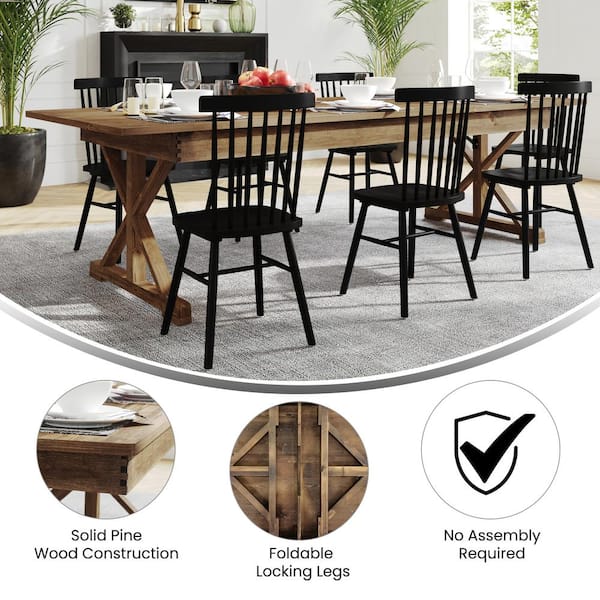The image is an advertisement showcasing a medium to dark brown, possibly oak or pine wood dining room table. The table features solid pine wood construction, foldable locking legs, and requires no assembly, as highlighted in three circular close-up images at the bottom of the image. The top two-thirds of the image depict the table fully assembled, surrounded by six black wooden chairs and staged with cutlery and a bowl of apples, set against a modern minimalist interior. The room features a sleek black fireplace, large windows, potted palms, and a stylish gray floor. A shield with a black check mark emphasizes the "no assembly required" feature.